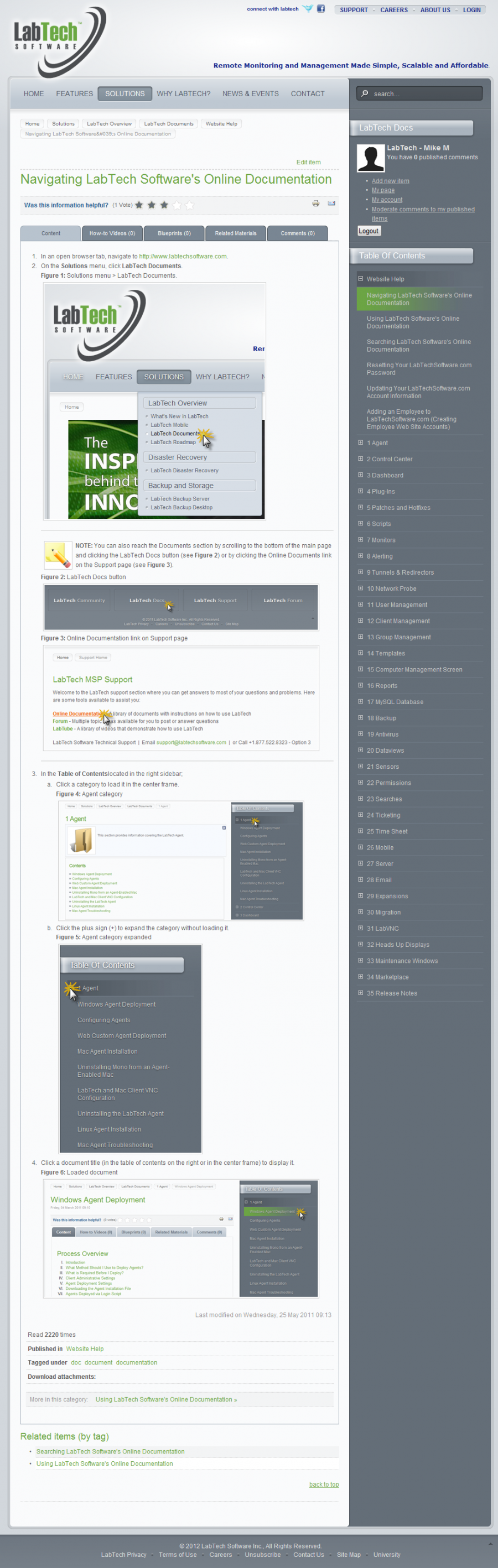This image is a screenshot of a webpage featuring a somewhat dated design, likely from around 2015 to 2017, or possibly earlier. At the very top left of the page, the company name "Lab Tech" is prominently displayed alongside its logo. "Lab" is written in a dark gray font, while "Tech" uses a green font. Circles or half-circles surround the word "Tech," lending it an appearance reminiscent of Saturn's wings.

The top header has a silver-gray background. Although the text within the top menu is too small to read, it is evident it contains several items. On the right side of the page, there is a sidebar with a bluish-gray background, filled with numerous items in white font, none of which are legible due to the small print.

At the top of this sidebar, there is a white square icon, likely indicating user account or profile access. The main background of the page on the left side is predominantly white. There is an additional menu with unreadable items due to the small font size. Below this menu, a smaller image appears to capture the top corner of the webpage, showcasing the "Lab Tech" logo again with some items listed underneath.